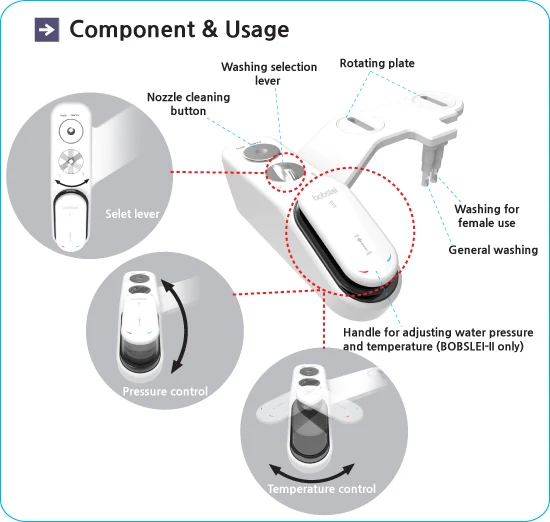This image is a detailed screenshot outlining instructions for using a specific gadget. The entire image is framed by a thin blue border with a white background. 

**Top Left Corner:**
- A small navy-colored square featuring a white right-pointing arrow, followed by the text "Component Usage."

**Main Section:**
- Central Gadget: A white device with a prominent flap and two circles on top. This gadget has an arm extending out, also white, featuring two disc-like holes.
- Below the arm, there are two small tubes protruding.

**Detailed Annotations (with circular zoom-in views and labels):**
1. **Top Left Circle:**
   - Features an alternate view of the gadget, labeled "S-E-L-E-T lever" (likely a typo for "Select lever").
   - An arrow indicates the lever's movement direction (left and right).

2. **Middle Left Circle:**
   - Positioned to the left of the central image, labeled "Pressure control."
   - A black arrow indicates adjustment directions (up and down).

3. **Bottom Circle:**
   - Located at the bottom of the screen, labeled "Temperature control."
   - An arrow shows the adjustment direction (left and right).

**Detailed Labels on the Gadget:**
- **Top Circles:**
   1. Labeled "Nozzle cleaning button."
   2. Labeled "Washing selection lever."
   
- **Front Flap Area:**
   - Red dotted line circle around this part with a label indicating "Handle for adjusting water pressure and temperature" (specific to "B-O-B-S-L-E-I-I-I only").
   
- **Arm Slots:**
   - Blue dotted lines point to these, labeled "Rotating plate."

- **Two Small Tubes at the Bottom:**
   - Right tube labeled "Washing for female use."
   - Left tube labeled "General washing."

**Top Circle:**
   - Red dotted line circle and a line pointing to the primary image, enhancing focus on that area.

This is a comprehensive visual guide to using the gadget, showcasing each part, its function, and how to operate it efficiently.